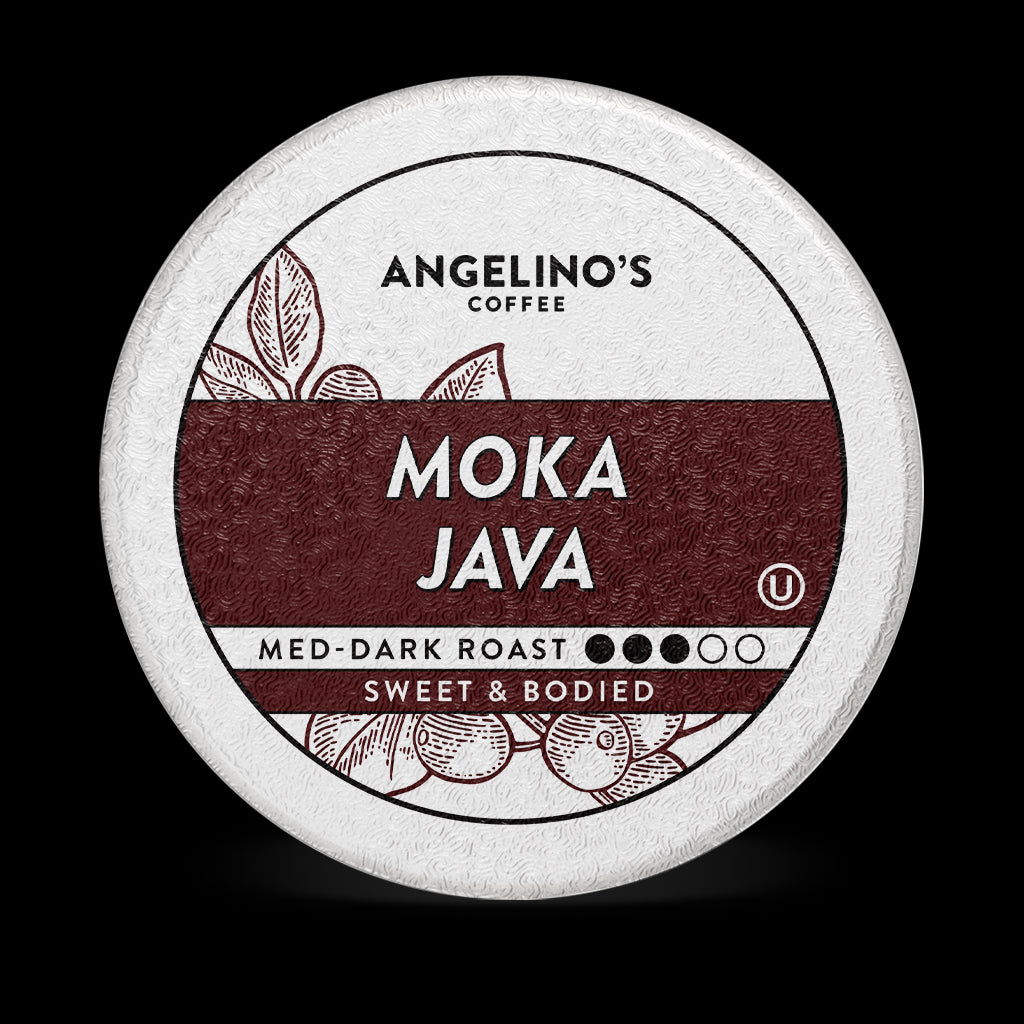The image is a color photograph in a square format, showcasing a top-down view of a Keurig K-cup coffee pod against a black background. The K-cup’s label is predominantly white with a detailed design. At the top, there is black text that reads "Angelino's Coffee." Beneath that, a horizontal maroon banner features the text "Mocha Java" in white. Below the banner, three out of five circles are filled in black, indicating a Medium Dark Roast, and the text "Sweet Bodied" is displayed. The label also includes graphics of coffee beans and a leaf towards the bottom, enhancing its visual appeal. The image employs a Photographic Representationalism style, capturing the detailed realism of the product.